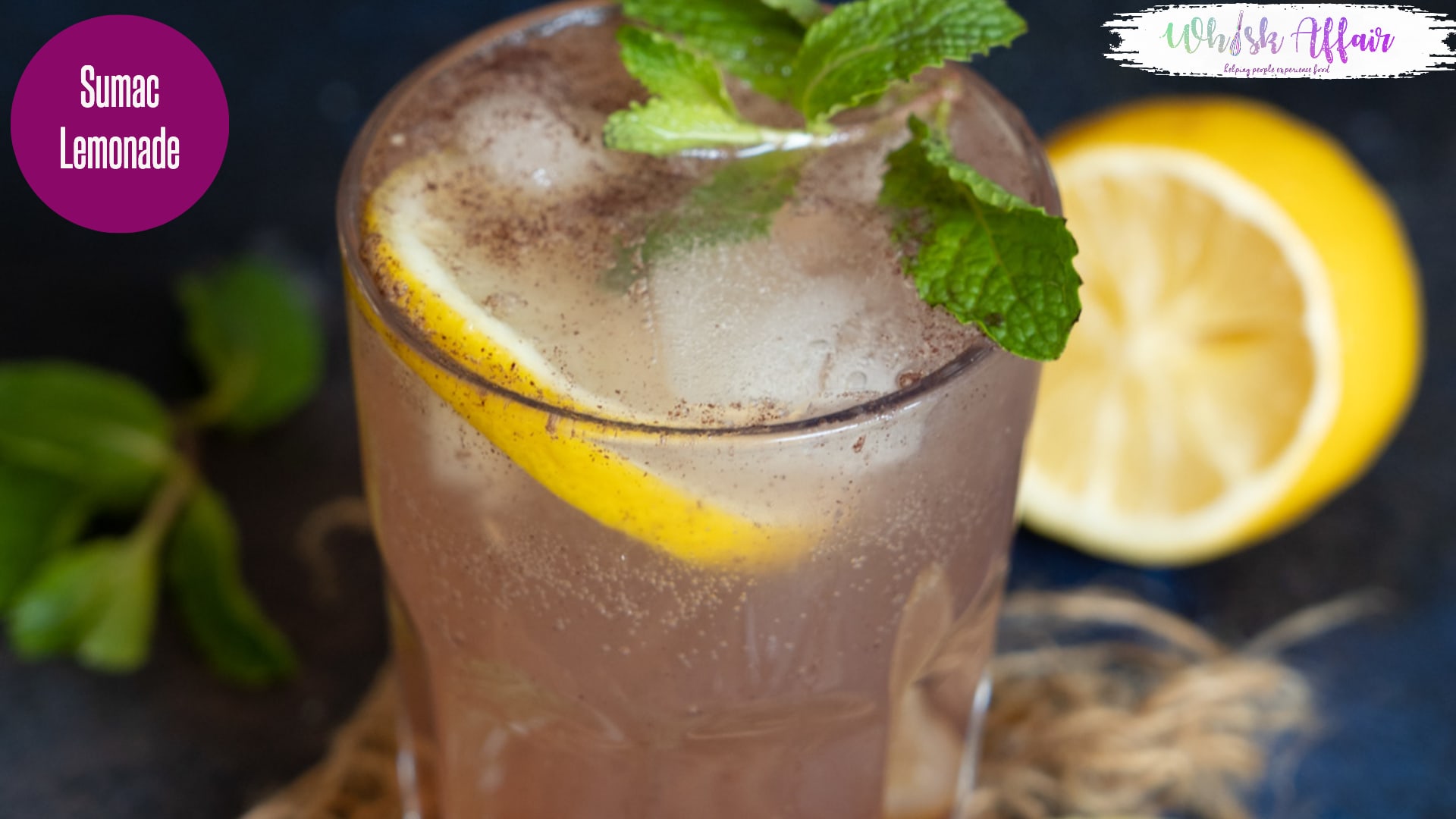This close-up photo showcases a glass brimming with iced Sumac Lemonade. The light pink, frosty beverage is adorned with ice cubes, a slice of lemon, and sprigs of mint at the top. The glass is sharply in focus, while the background remains blurred. Nearby, to the right, rests a lemon with a slice removed, and to the left, additional sprigs of mint lie scattered. In the upper left-hand corner, a purple circle with white letters reads "SUMAC" and "lemonade." In the upper right-hand corner, a cream-colored label bordered in white displays the phrase "Hoosh Affair." A small brown, basket-like dressing decorates the base of the glass, adding to the overall aesthetic appeal of this refreshing drink.